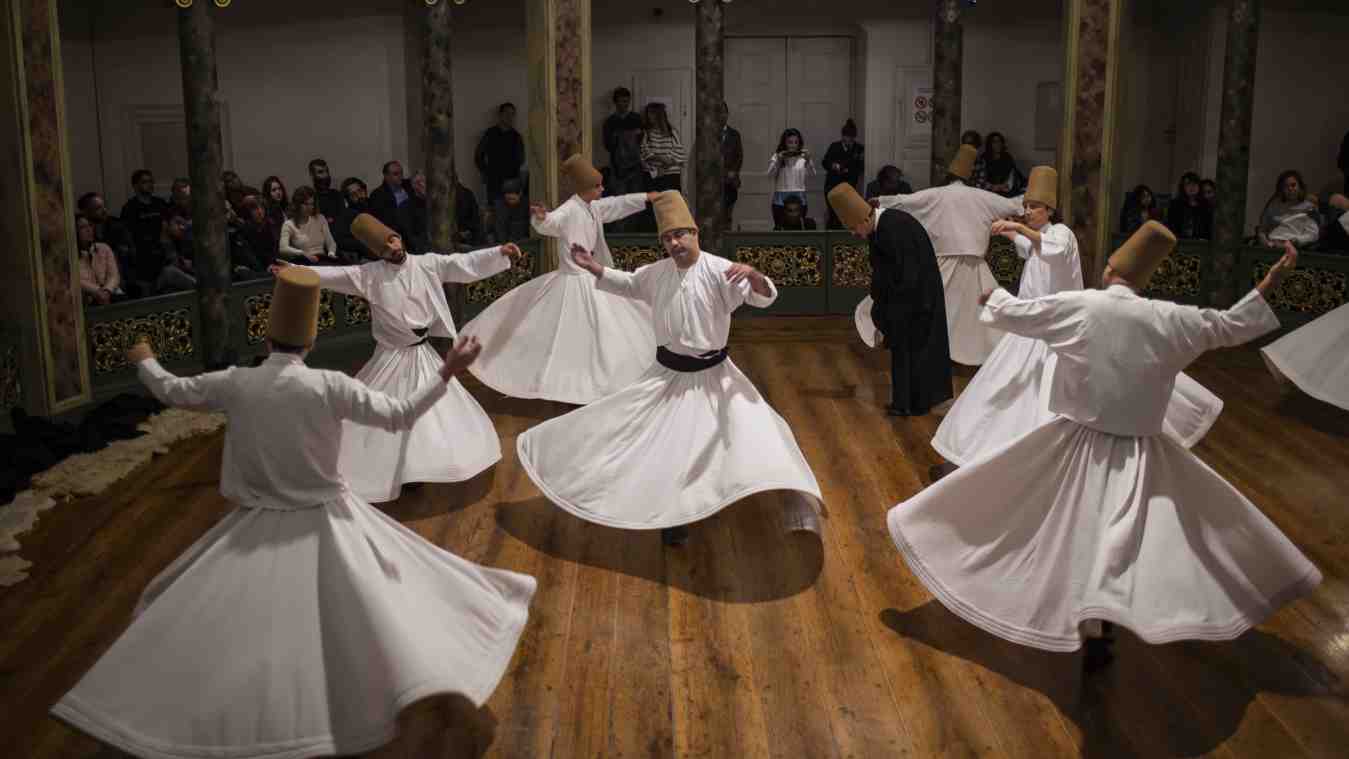The image captures a vibrant dance hall teeming with cultural flair. Nine men are dressed in exquisite traditional attire, featuring flowing white robes cinched with black belts at their waists. These garments accentuate their movements as they dance energetically on a circular wooden floor. Adding to their ensemble, the men don cylindrical light brown caps and white shirts, creating a striking contrast with their garments.

Amidst the dancers, one man stands out in a black robe, with a similar brown cap, positioned centrally and appearing reflective, not participating in the dance. 

The scene is framed by an array of spectators who encircle the dance area, cheering and observing the lively performance. Behind the crowd, a low green wall segmented by both round and square wooden pillars separates the dance floor from an elevated gallery area. 

Further back, a whitish-gray wall with multiple doors adds depth to the room, suggesting exits beyond the gallery. The overall atmosphere suggests a celebratory event, rich in tradition and communal participation.